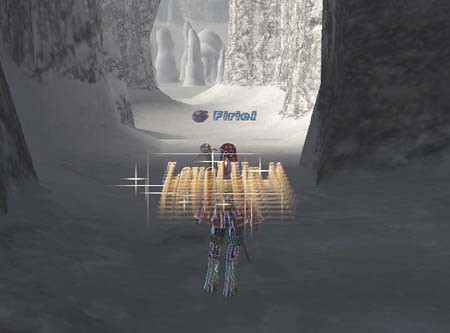In this vivid video game scene, a character is depicted from behind, standing resolutely within an icy, snow-laden cave. The character is garbed in an intricately detailed suit of armor, resplendent with red and brown hues, imparting a sense of strength and preparedness. Grasped firmly in their hand is a formidable staff or weapon, hinting at their combative potential. Ahead of the character glows a shimmering golden shield-like aura, suggesting an active magical or protective power being employed. The cave itself is rugged, with walls encrusted in snow and ice, and a pathway that meanders deeper into the mysterious, chilly expanse. Over the pathway, a blue sign with white lettering spells out "Fyriel," adding a touch of lore to the environment. The overall atmosphere exudes coldness, perfectly aligning with the icy cave setting, while the character's outfitting underscores their readiness for imminent adventure or conflict.